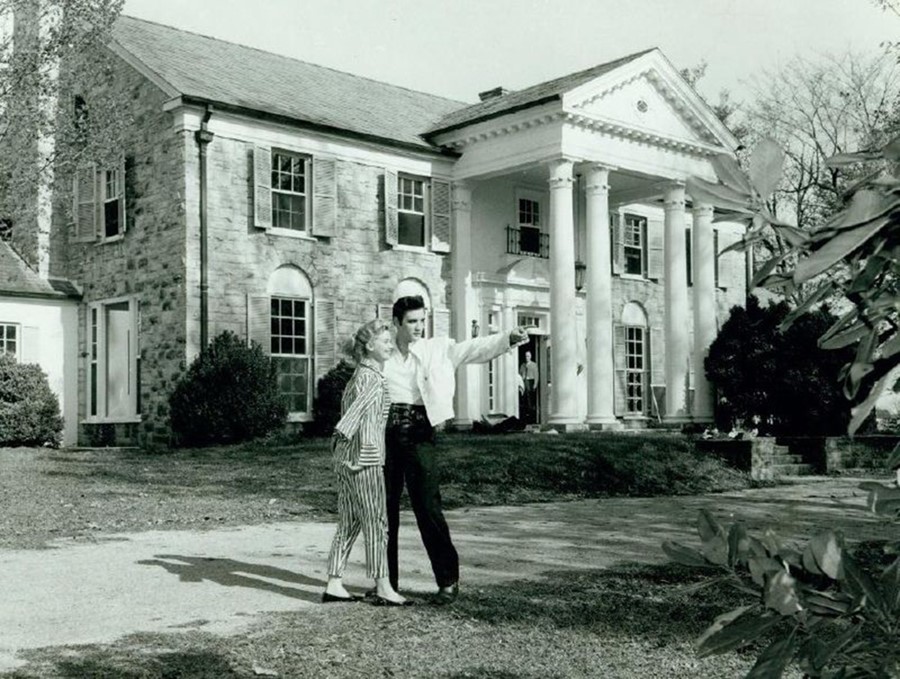This black-and-white photograph captures Elvis Presley standing in front of Graceland, his iconic home, during the daytime. Elvis is dressed sharply in a white short jacket and black pants, which feature buckles instead of a traditional fly. His left leg is slightly bent, and he is pointing into the distance with his left hand, a smile brightening his face. Beside him stands a woman, who is not Priscilla Presley. She is smiling and outfitted in a striped pantsuit with flat shoes. The woman’s attire, including striped pedal pushers, might look like pajamas to some. Behind them, Graceland’s stately facade is visible, complete with large white pillars, arched windows, and open shutters. The shadows of Elvis and the woman stretch out behind them, adding depth to the scene. Additionally, an elderly man, possibly a butler, stands in the doorway, observing the interaction. The surroundings are lush with trees and shrubbery, framing the house and adding to the grandeur of the snapshot.